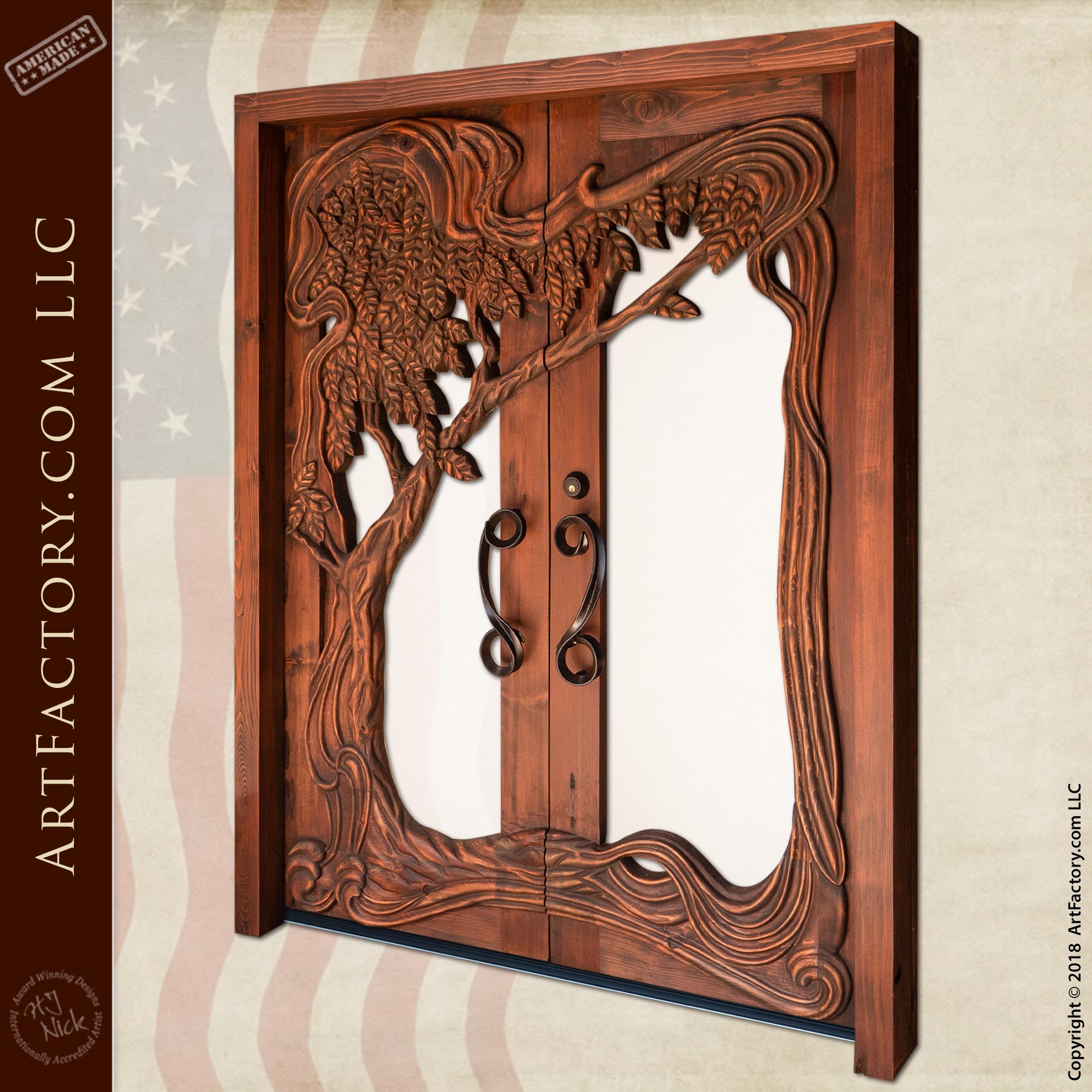The image features a meticulously hand-carved, medium-toned, reddish wooden double door, possibly acting as a front or French door. Each door has a decorative black scroll handle, with a key lock situated above the right handle. Dominating the design is an intricately carved tree, predominantly on the left panel, with its branches and leaves extending gracefully onto the right panel. Framing the doors is a narrow brown border, and the space within the doors appears white, possibly indicating an absence of glass. The background showcases a beige hue with an American flag print on the left side. Alongside this, text reads "ArtFactory.com, LLC," "American made," and mentions H J Nick, an award-winning, internationally accredited designer. A watermark in the bottom right corner denotes "Copyright 2008, ArtFactory.com, LLC."